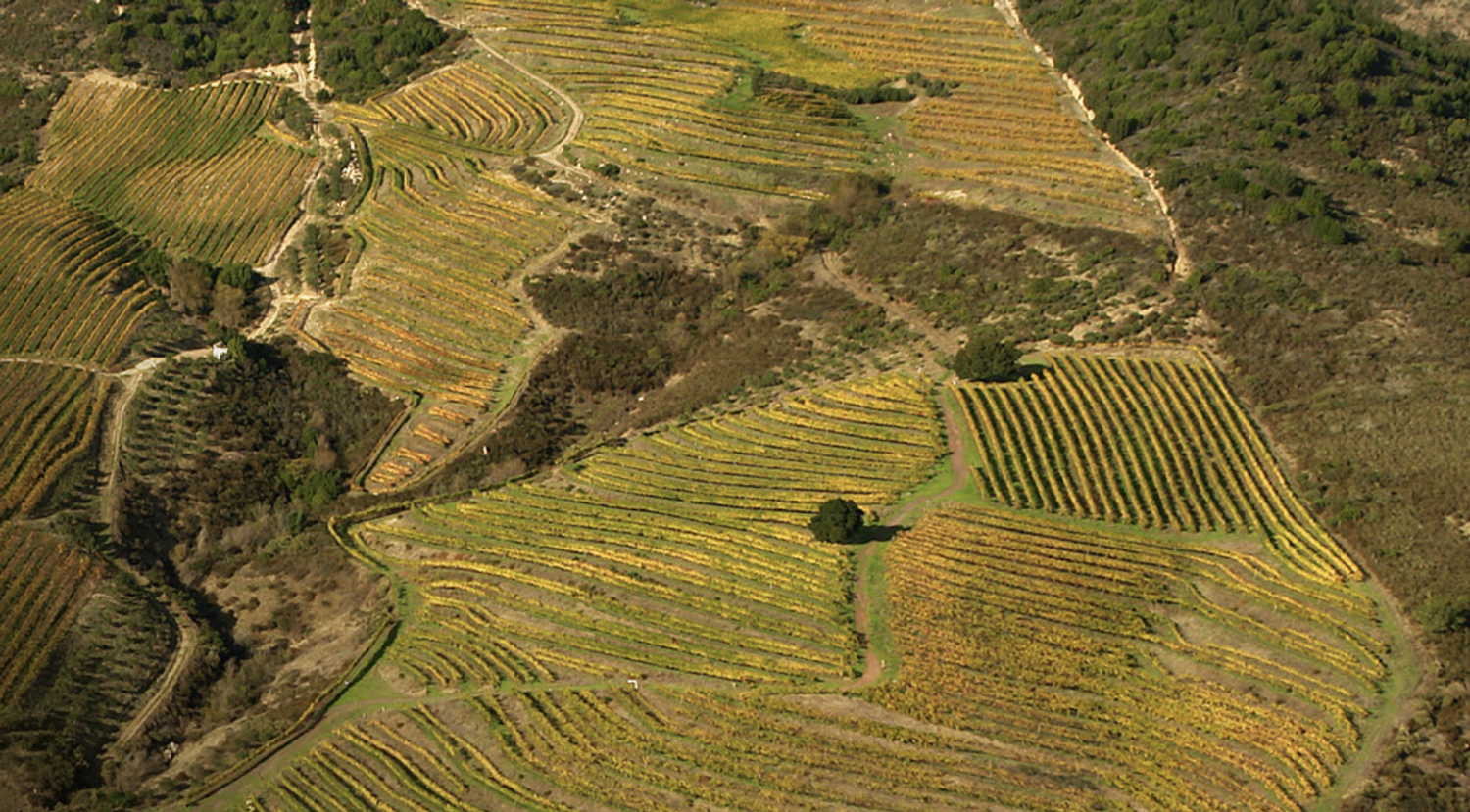The overhead, landscape-oriented color photograph captures an intricate patchwork of farms nestled into mountainous terrain. The central focus is a network of furrowed fields with rows of crops predominantly adorned with yellow flowers. These rows form irregular, zigzagging patterns across the hillsides. Prominent in the middle of the image is a distinctive triangular patch of barren land, characterized by brown brush and dirt. A noticeable green bush is situated near the center, amidst the cultivated areas. A winding road carves its way through the farms, beginning on the left, weaving rightward, then looping back up across the fields. The far right of the photograph shows rolling, vacant mountain lands with a blend of brown brush at the base and green trees atop. The scene is meticulously detailed, offering a snapshot of agricultural life set against a backdrop of natural rugged beauty, captured from an aerial perspective.